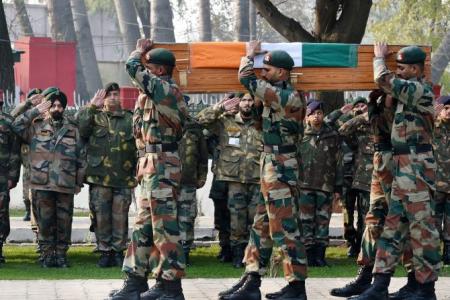The image depicts a solemn, outdoor military funeral procession for a foreign military member. Six Iraqi soldiers, dressed in green, tan, and brown camouflage uniforms with green berets, are carrying a wooden casket draped with an Iraqi flag, distinguished by its orange, white, and green colors. The soldiers are marching in step, each with their right foot forward and left foot back. In the background, additional military personnel are lined up in columns or rows, saluting the casket. Among them, most are wearing berets, while a few are wearing kibosks or turbans. The setting is grassy, with trees visible, adding to the serious and somber atmosphere of the funeral.